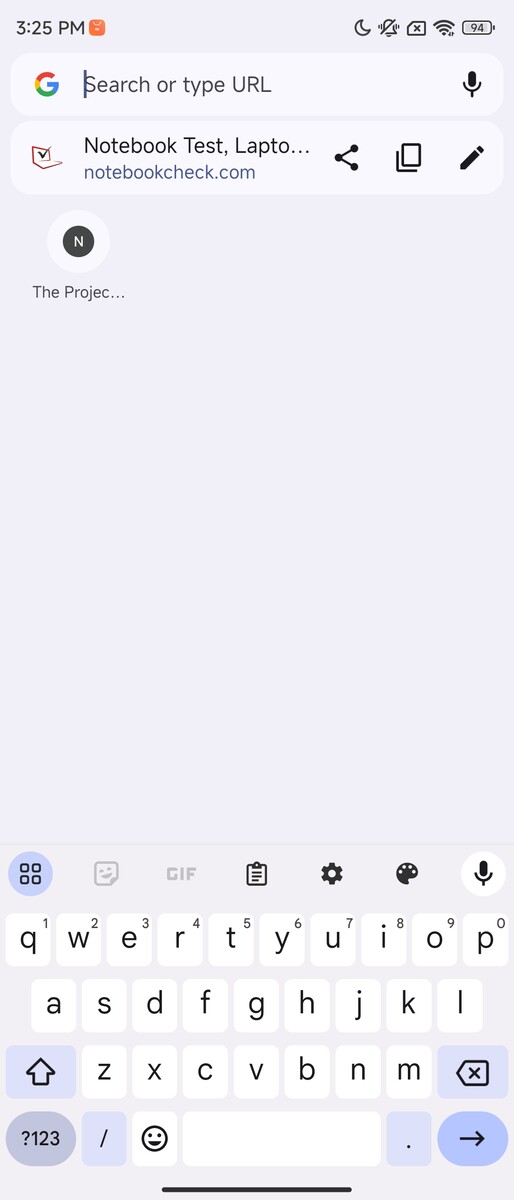The image features a Google search bar prominently displayed at the top, adorned with the colorful 'G' Google logo on the left side. Within the search bar, the text "Search or type URL" is visible, and a microphone icon is situated on the right end of this input field. 

Beneath the search bar, a section lists various terms including "notebook," "text," "laptop," and "Lollipito," followed by three colons. To the left of this text block is an image of a laptop. On the right side of this section, there are icons for sharing, a document page, and a pencil.

Further down, there's a white circle with a black center, which contains a prominent white letter 'N'. Below this icon, the text "the projec..." is partially visible. This entire segment is set against a gray background that occupies most of this part of the screen.

At the bottom of the image, a virtual keyboard is displayed. It features keys labeled with the letters Q, W, E, R, T, Y, U, I, O, P, A, S, D, F, G, H, J, K, L, Z, X, C, V, B, N, and M. Additionally, there are function keys including an up arrow, a space bar, and a key with a smiley face at the bottom. On the far left of the keyboard is a gray key marked with a question mark and "1 2 3". To the right, a blue button with a black right-facing arrow is visible.